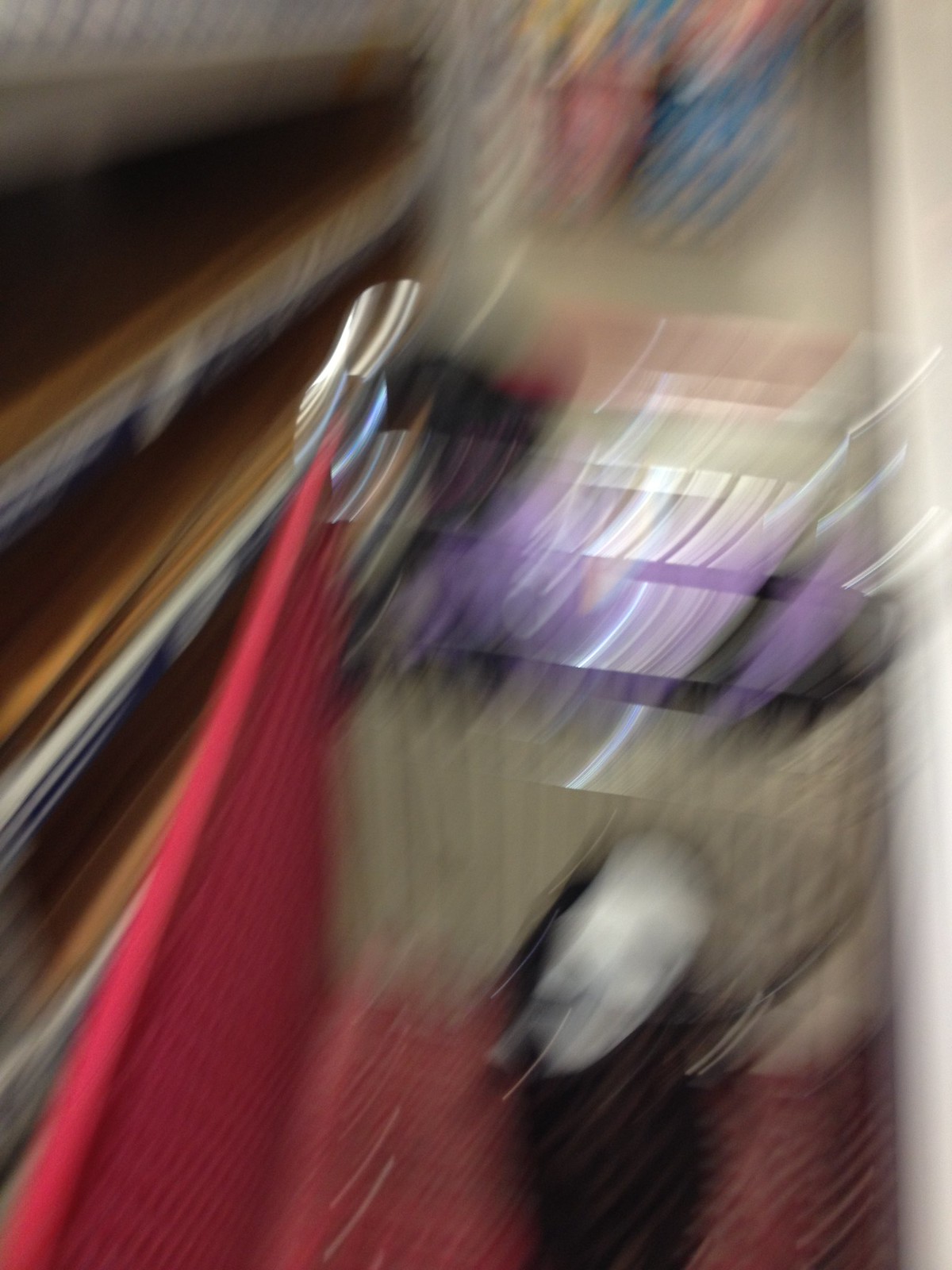In this blurred and dynamic image, a red shopping cart is prominently featured, seemingly in motion as if someone was running with it. The cart’s basket, vividly red, contains a few indistinct objects. One object appears to be predominantly white with a black cloth or texture beneath it, though the exact nature of this item is unclear due to the blurriness. Additionally, a hint of something purple is visible in the section of the cart usually designated for a child's seat. There are no people visible in the image, and the scene appears to be set in a standard shopping aisle, adding to the everyday context of the moment captured.